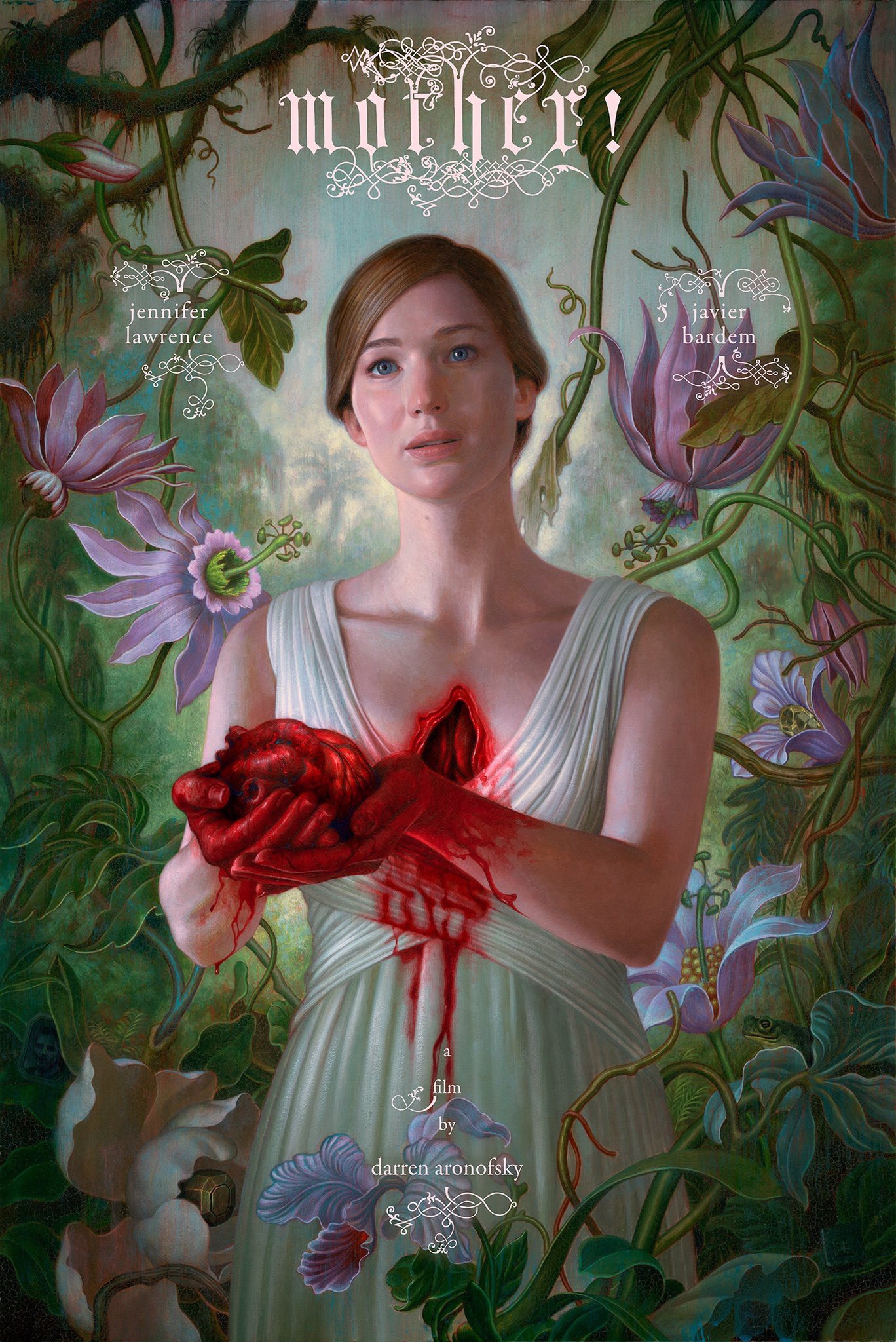The image appears to be a detailed poster for the film "Mother!" directed by Darren Aronofsky. At the top of the poster, the title "Mother!" is prominently displayed in an elaborate font. Below the title, the names of main actors Jennifer Lawrence and Javier Bardem are listed. The centerpiece of the image is an illustration of Jennifer Lawrence, standing in what seems to be a lush garden or forest surrounded by green leaves, purple sunflowers, and vines. She has light brown hair pulled back and is dressed in a pristine white dress smeared with blood. A gruesome, gaping wound is visible in the center of her chest, from which blood is flowing down, staining her dress. She is holding a human heart in her outstretched, blood-streaked hands, with blood dripping down her wrists. This striking and surreal imagery is further emphasized by the detailed background of intertwining flora, adding to the ethereal and haunting atmosphere of the poster. At the bottom, it states "a film by Darren Aronofsky," completing the darkly thematic promotional artwork for the film.